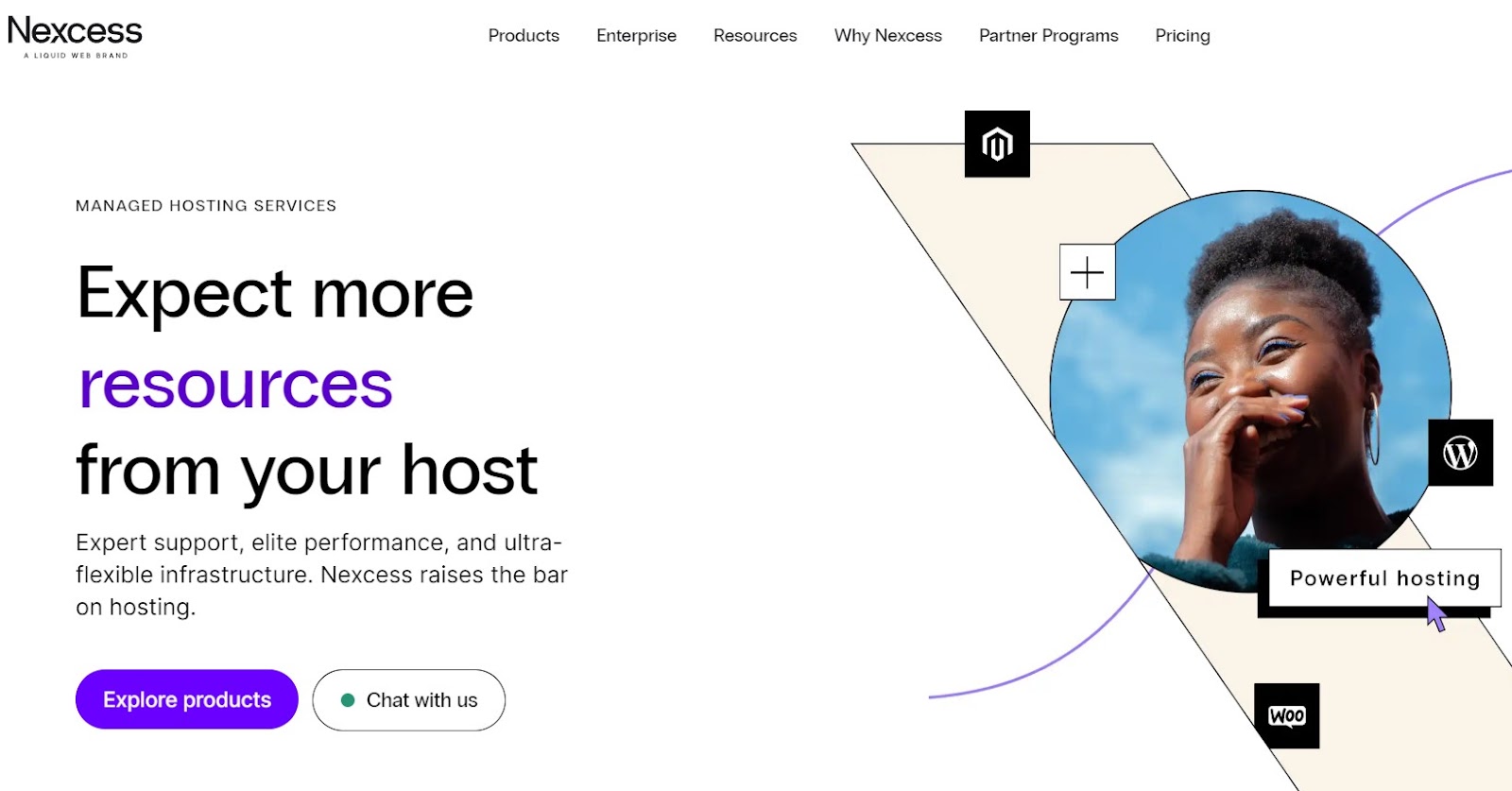This image displays a website by Nexcess, prominently indicated by the company's name in black letters in the upper left corner, spelled "N-E-X-C-E-S-S." To the right, there's a navigation menu with clickable options: "Products," "Enterprise," "Resources," "Why Nexcess," "Partner Programs," and "Pricing." 

Beneath the menu, there's a picture of a smiling woman with her hand partially covering her joyous expression. Directly below her image, a prominent clickable rectangle reads "Powerful Hosting," accompanied by a clickable mouse arrow icon. 

On the left side of the image, there’s a small heading that says "Managed Hosting Services." Larger text below this declares, "Expect More Resources from Your Host," with the word "Resources" highlighted in blue. A subheading in smaller letters lists key benefits: "Expert Support," "Elite Performance," and "Ultra-Flexible Infrastructure," along with the statement, "Nexcess raises the bar on hosting."

At the bottom, there are two more clickable areas: a blue button labeled "Explore Products," and a green button with a dot that reads "Chat With Us."